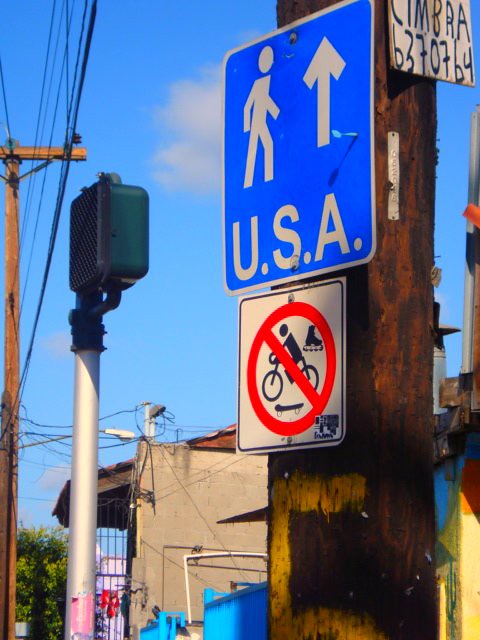The photograph, oriented vertically, captures a quintessential back street in the USA. Dominating the right side of the image is a telephone pole, its top and bottom out of frame, bringing the focus to its various signs. A prominent blue sign reads "Walking USA," accompanied by a white sign below that prohibits skating and bike riding, marked by red circle symbols. Higher up, a wooden sign displays "Simbra B370764."

In the background, the rear facades of various buildings are visible, featuring diverse architectural styles and colors. To the left of the main telephone pole, a speaker is positioned, and further left, at the very edge of the image, another telephone pole appears, with connecting wires stretching into the distance.

The scene is dotted with numerous security cameras or lights, adding an element of surveillance. A secondary focal point is a building with slightly olive-toned bricks, situated left of the main telephone pole, while behind it, another structure painted in yellow with blue and orange accents adds a splash of color.

Occupying more than half of the upper portion of the frame, the blue sky with wispy clouds indicates a clear daylight setting, adding a serene backdrop to this urban landscape.